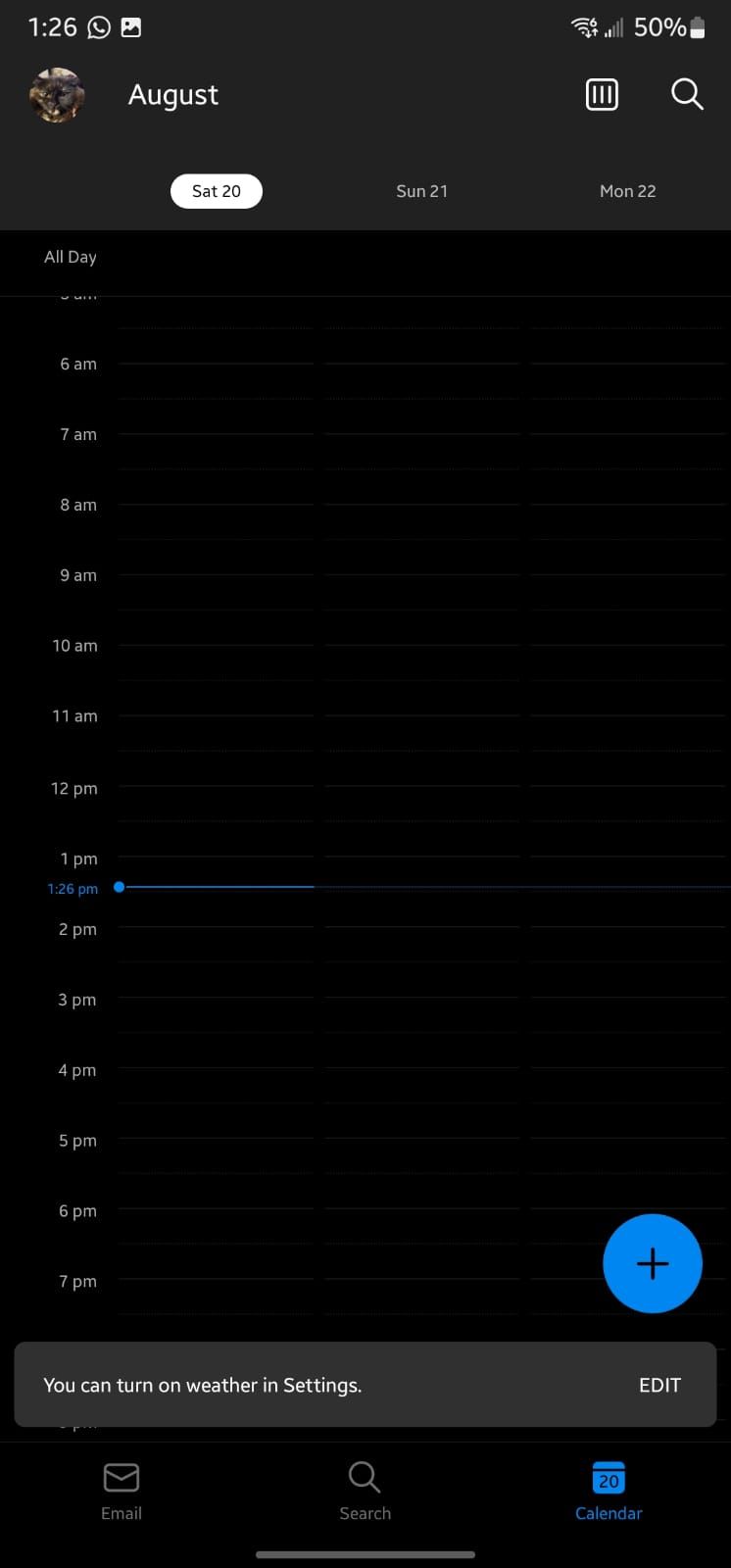This is a detailed screenshot captured on a smartphone, showcasing a utility app interface with a gray and blue color scheme. At the top of the screen, the user interface displays the time as 1:26 PM, with notifications from WhatsApp and the image gallery, a Wi-Fi symbol, mobile data icon, and a battery level at 50%.

The main content area is labeled "August" at the top, featuring a small profile picture on the left and a menu icon (three horizontal bars) and a magnifying glass icon on the right. Below this heading, there’s a calendar interface that displays three specific dates: Saturday 20th, Sunday 21st, and Monday 22nd of August. The calendar adopts a vertical layout, presenting time slots from 6 AM to 7 PM. Highlighted at 1:26 PM is an event marked with a distinctive blue dot and a blue line extending from it.

Additionally, there's a prominent blue circle with a plus sign positioned to add new events. A pop-up notification at the bottom of the calendar view suggests enabling weather updates in the settings, with an "Edit" option next to it.

Finally, the bottom of the screen features three tabs: "Email," "Search," and "Calendar," with the calendar tab highlighted in blue to indicate it's the current active section.